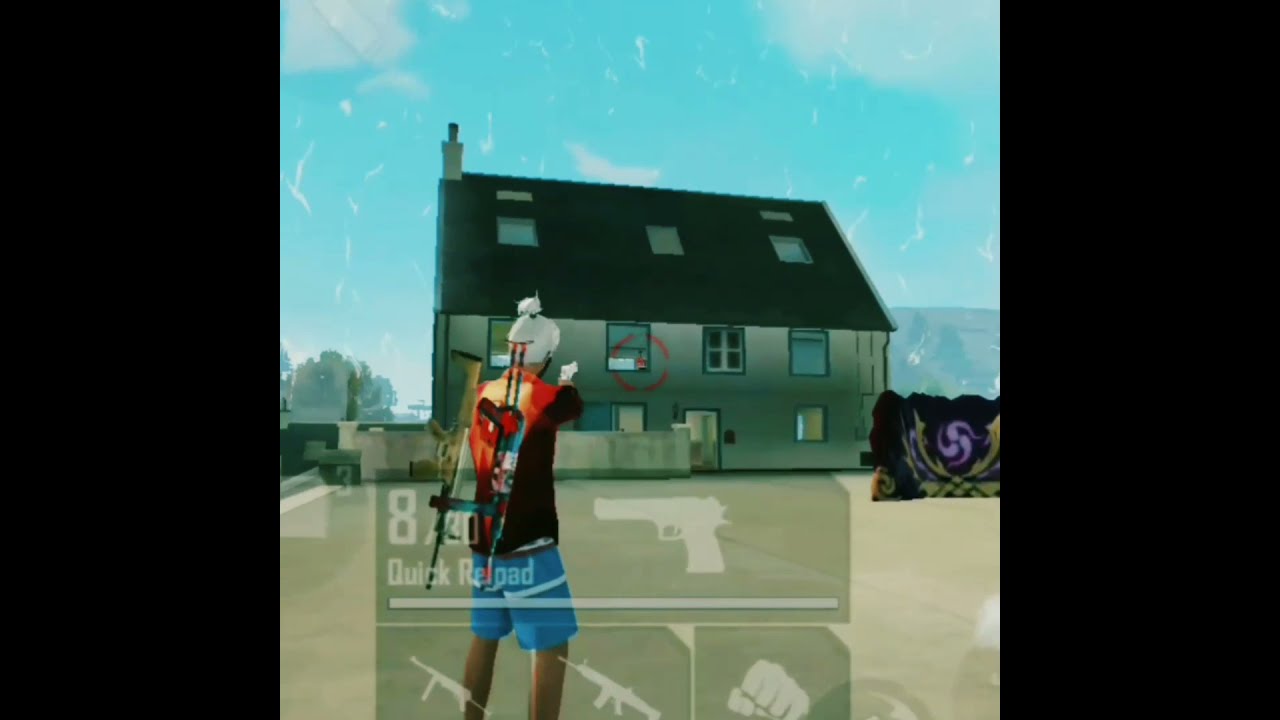The image is a detailed screenshot from a first-person shooter video game, capturing a moment where a character is aiming a gun at a house. The main character, seen from the back, has white hair tied in a bun and a tan complexion. He is equipped with a handgun, with additional weapons on his back – one gun is green, brown, and tan, while the other is red, blue, and white. He is dressed in a red shirt with yellow accents and light blue shorts. The game interface is visible, showing an 8 out of 30 ammo count and a "Quick Reload" option, along with icons for various weapons including a fist for melee combat.

The setting features a house with gray siding, a black roof, and windows covered with gray curtains. A red aiming reticle indicates the target on the house, specifically near a window. The scene is set outdoors, under a bright blue sky with white clouds, and green trees are visible in the background, along with a distant mountain range. The ground in the foreground is light beige with a gray wall. On the right side of the image, there's a flag-like object with a purple and gold design. The image also has thick black strips on both sides, possibly framing the screenshot.